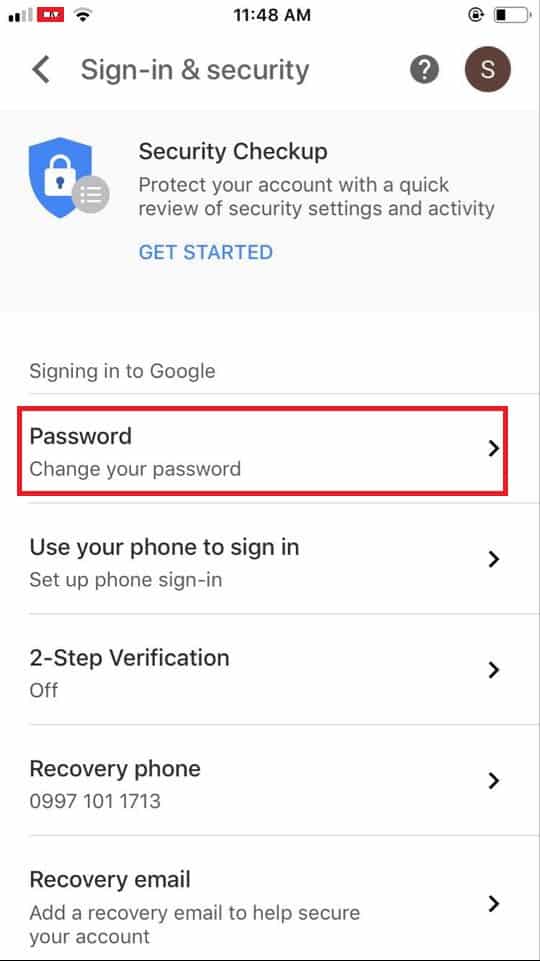A screenshot of a smartphone display shows specific details at 11:48 a.m., with the status bar indicating two out of four signal bars and about a quarter of battery life remaining. The screen presents a "Sign in & Security" section prompting the user for a security checkup with the message: "Protect your account with a quick review of security settings and activity." Below this prompt is a "Get Started" button.

The subsequent part of the screen features several rectangular sections, each set against a white background and separated by a light gray line that almost spans the screen width but not completely. Each section has a title in black font and a description in gray font beneath it:

1. **Password**
   - **Change your password**
   - (Accompanied by a right-facing 'greater than' symbol)
   
2. **Use your phone to sign in**
   - **Set up phone sign-in**
   - (Accompanied by a right-facing 'greater than' symbol)
   
3. **Two-step verification**
   - **Off**
   - (Accompanied by a right-facing 'greater than' symbol)
   
4. **Recovery phone**
   - **0997 101 1713**
   - (Accompanied by a right-facing 'greater than' symbol)